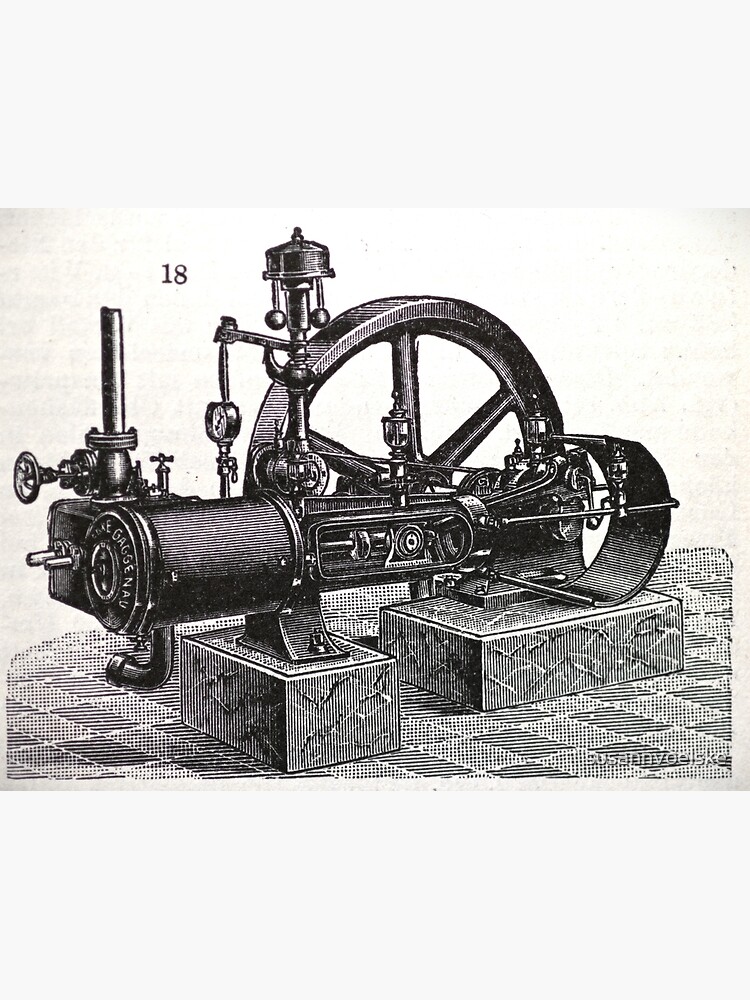This black and white magazine-style drawing features a detailed depiction of an old-fashioned steam engine, characterized by its intricate mechanisms and industrial elements. The machine, seemingly made of metal, is mounted on two sturdy blocks and positioned on a checkerboard-patterned floor. The foreground prominently displays a large enclosed piston labeled “gauge,” which leads to an open cylinder revealing internal pistons. Above this assembly, a pipe extends to a dome-shaped lid with two balls suspended from it, indicative of a pressure release mechanism. Behind the piston is a big metal wheel, adding to the complexity of the machine. Various pipes and canisters are connected sporadically throughout the device, highlighting its intricate design. The entire scene is rendered in black and white tones, with a slightly dingy cream background, lending an antique ambiance to the illustration. Notably, the number 18 is inscribed in the top left-hand corner of the image.